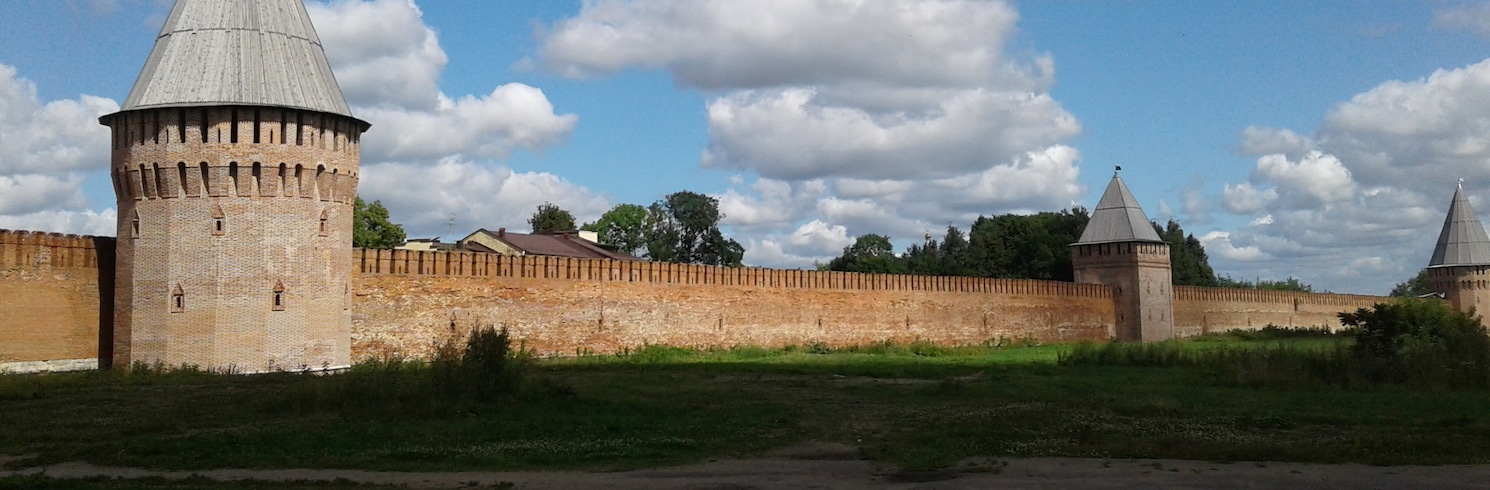The photograph showcases a sprawling ancient castle wall that runs the entire width of the rectangular frame, dominating the scene. This formidable stone wall, tan to brown in color, features three distinct towers: the first is round, the second is square, and the third has a unique rounded shape on its right side. Topped with pointy, triangular roofs, the towers evoke an image of historical fortification. The vibrant green lawn in the foreground, sprinkled with some bushes, contrasts with the stone wall's earthy tones. Behind the wall, a maroon-roofed building peeks through, and amidst the background foliage, trees can be seen. The sky above is a clear, soft blue with harmless, fluffy white clouds, completing this picturesque outdoor scene.